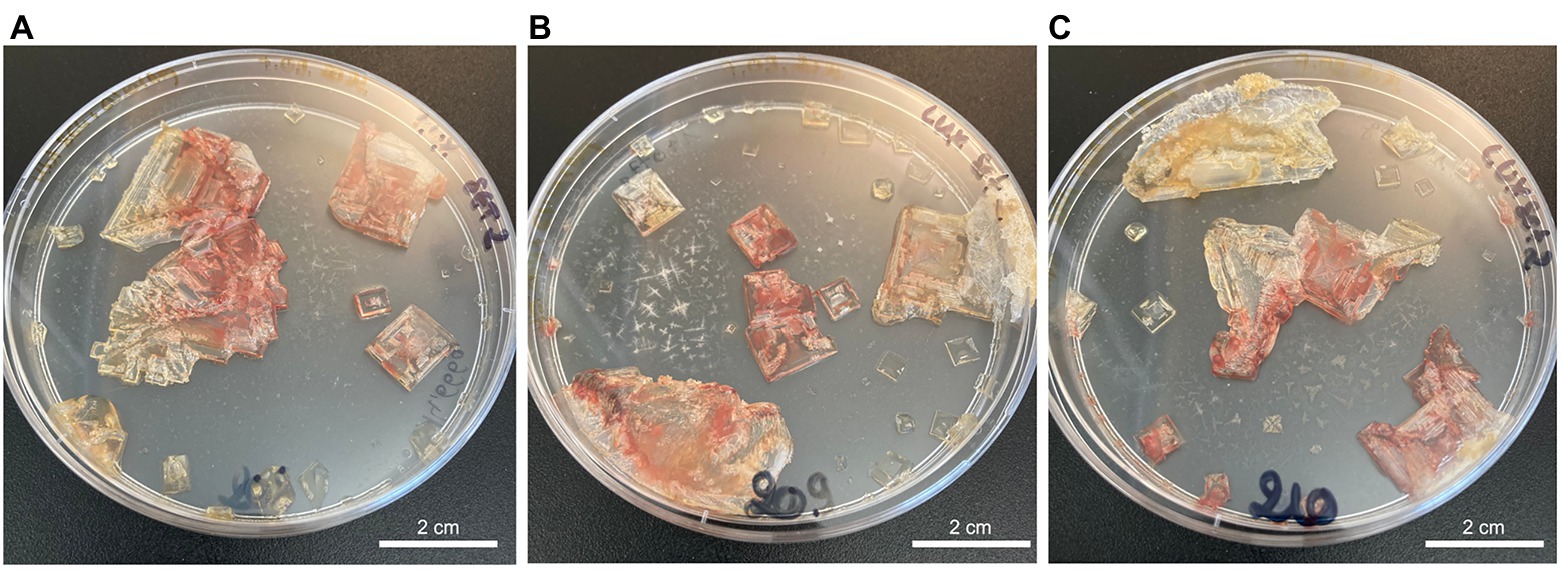The image depicts three different Petri dishes labeled A, B, and C, and numbered 208, 209, and 210 respectively. Each Petri dish measures two centimeters in diameter and is set against a dark gray background. The dishes are clear, round, plastic containers with identifiable writing on them. Petri dish A is filled with variously sized beige and red bacteria colonies, including larger, skin-like pieces and smaller square-shaped bacteria. Petri dish B contains fewer but similarly arranged colonies, predominantly featuring more square-shaped bacteria pieces. Petri dish C shows a transformation, where some of the square bacterial segments have become more skin-like, while the remaining squares have reduced in size. The Petri dishes, nearly filling up the squares they are set in, exhibit a gradient of bacteria density and types, changing visibly from A to C.